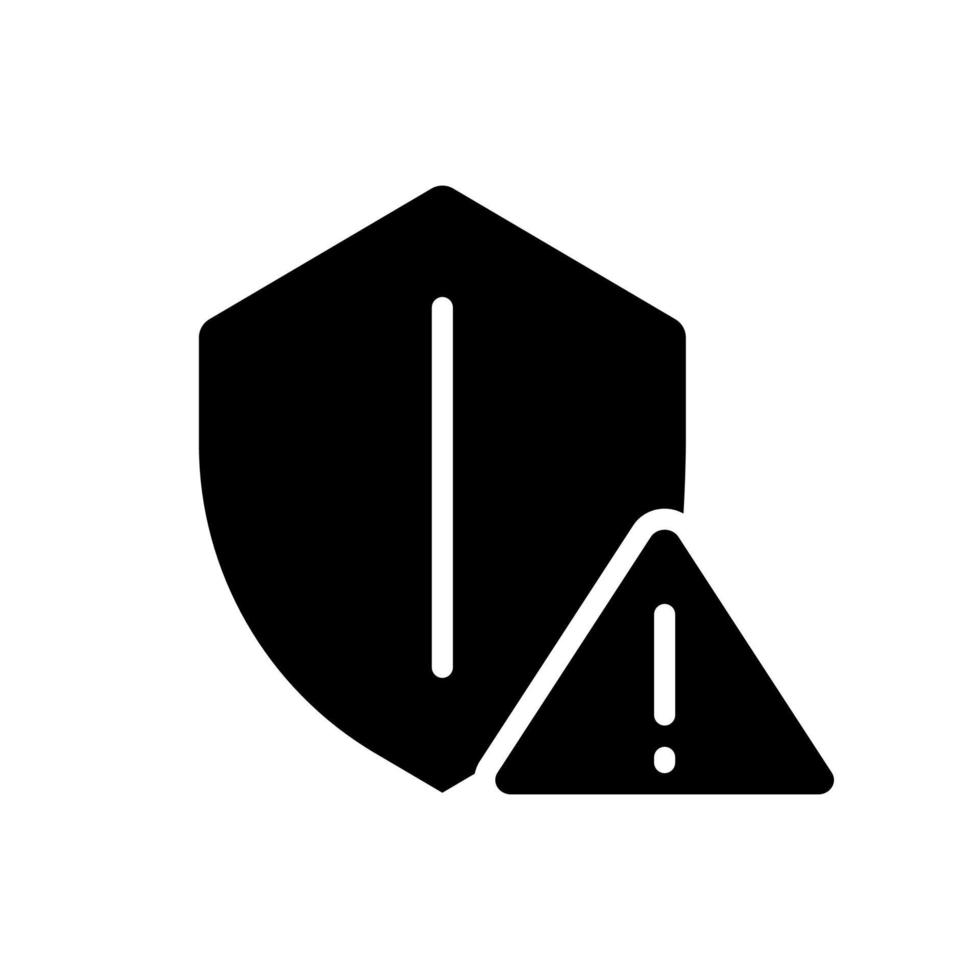The image features a simplistic black and white logo consisting of two overlapping elements against a white background. Central to the design is a black shield, reminiscent of a medieval shield, with a single, solid white line running vertically down its middle. Overlapping the bottom right corner of the shield is a smaller, black, equilateral triangle with a bold white exclamation mark in its center. The triangle, which is about one-third the size of the shield, serves as a caution symbol. A white outline distinguishes the overlapping area, ensuring both shapes remain distinct. Together, the shield and the caution triangle create a composite symbol that conveys a sense of warning or danger. The stark contrast between the black shapes and the white background emphasizes the design's simplicity and effectiveness, potentially making it suitable as a logo or safety warning icon.